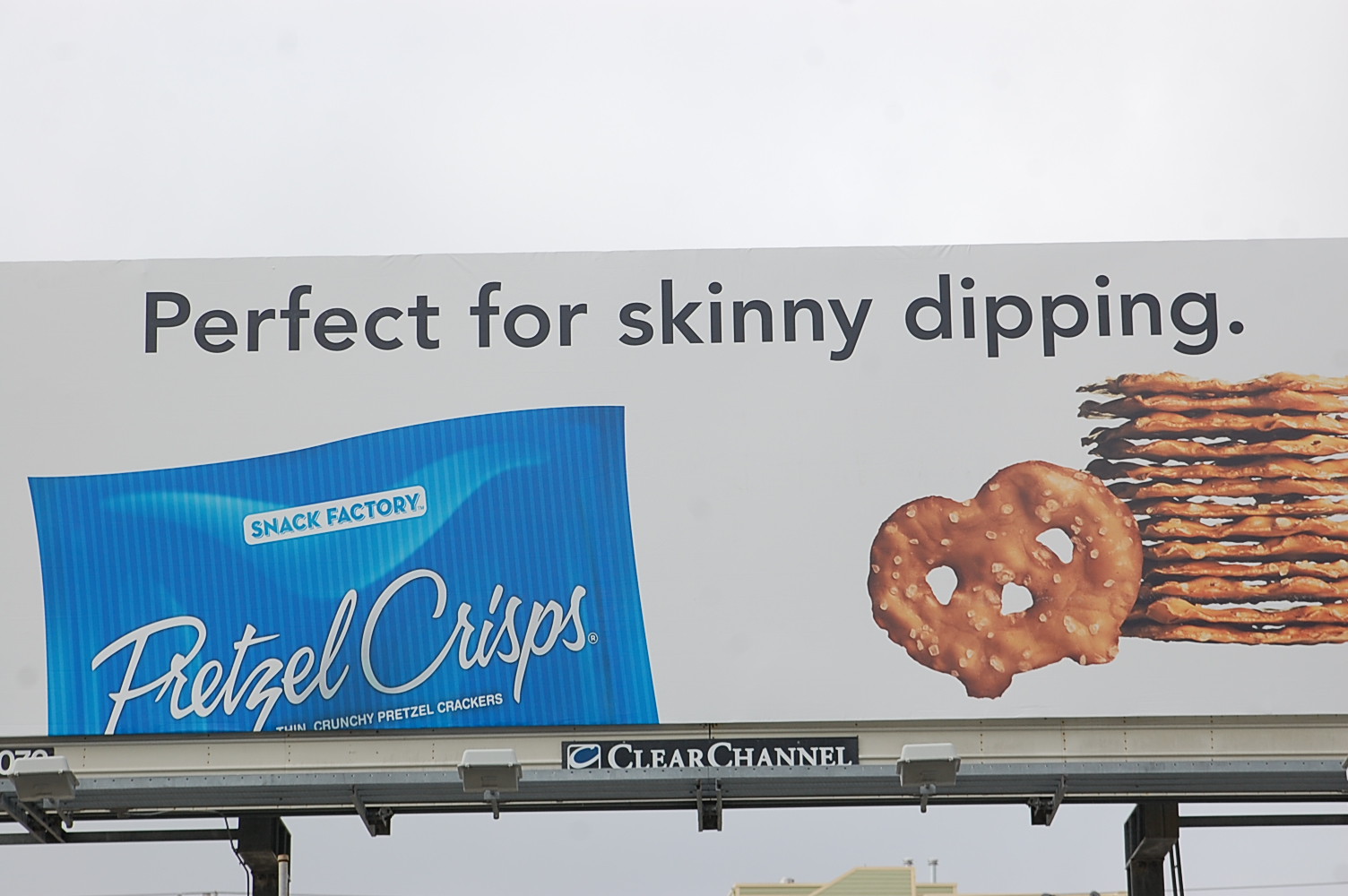The image showcases a large billboard prominently displaying an advertisement for Snack Factory's Pretzel Crisps. The billboard features a vivid blue bag of Pretzel Crisps, adorned with the brand's name in elegant cursive script. Below the bag, the phrase "Crunchy Pretzel Crackers" is clearly visible. The visual design includes a detailed picture of a single flat pretzel along with a small stack of pretzels beside it. The tagline "Perfect for skinny dipping" is creatively placed on the billboard, adding a playful touch. The billboard is equipped with lights at the bottom, designed to illuminate the advertisement, though they are currently turned off. The backdrop of the image reveals an overcast sky, casting a gray hue over the scene. At the bottom and center of the image, the top portion of another building is faintly visible, indicating an urban setting. The lower part of the billboard is marked with the "Clear Channel" insignia, identifying the advertising company responsible for the display.